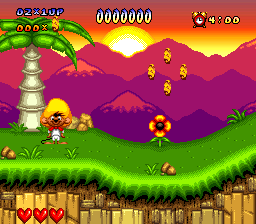The image is a screen from a 2D cartoon-like video game. The color palette is rich with browns, greens, yellows, purples, oranges, and reds. The scene is a cutaway landscape that reveals the subterranean layer, showcasing various shades of brown dirt and rocks. Above this earthy layer, lush green grasses in dark, middle, and bright green hues blanket the surface. Yellow-brown rocks and tufts of dark and light green grass add texture to the ground.

On the left side, a palm tree with a brown trunk and green fronds stands prominently. Nearby, a small mouse character dressed in a white outfit, red bow tie, and a yellow sombrero looks directly at the viewer. In the middle of the scene, a flower with a deep brown center and yellow and red petals adds a splash of color.

The background features a series of receding mountain ranges in dark purple, violet-pink, and red hues, set against a vibrant sunset. Some bees and possibly mushrooms or cocoons are scattered throughout the greenery. The top of the screen displays blue and yellow lettering and numbers, likely representing the game’s score, with a row of zeros and an alarm clock showing 4:00, indicating the remaining time to play. At the bottom, there are three colored hearts representing the player's life count.